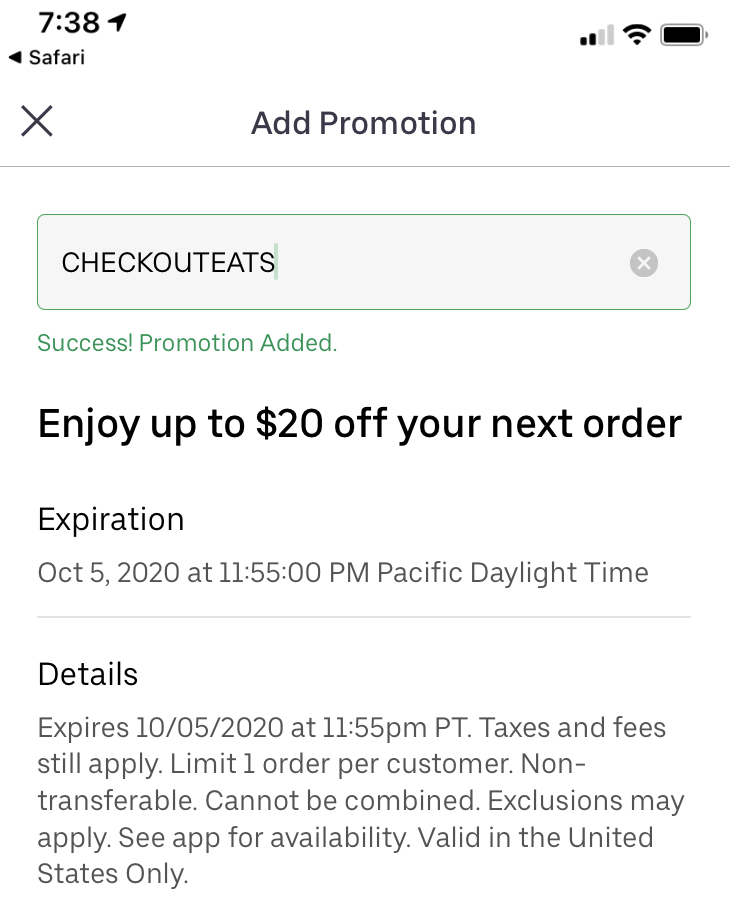**Detailed Caption:**

This image shows a smartphone displaying a webpage within the Safari browser. At the top of the screen, a timestamp reads 7:38, accompanied by a "Send or Share" arrow icon. Directly below, there is a navigation bar with a left-facing arrow labeled "Safari," followed by a "crossout X" icon. Centrally positioned is the text "Add Promotion."

In the upper right corner of the screen, there are icons indicating a strong Wi-Fi signal and a fully charged battery. Underneath these icons lies a search box containing the term "CheckoutEats," written as one word, with a blinking cursor at the end of the text. To the right of the search box is another "crossout X" icon.

The main body of the page displays a confirmation message, "Success! Promotion added." It announces that users can "enjoy up to $20 off your next order," with an expiration date of October 5th, 2020, at 11:55 p.m. Pacific Daylight Time.

The details section reiterates the expiration date and provides additional terms:
- Taxes and fees still apply.
- Limit one order per customer.
- Non-transferable.
- Cannot be combined with other offers.
- Exclusions may apply.
- See app for availability.
- Valid in the United States only.

This promotion is specifically for "CheckoutEats," allowing users to receive up to $20 off their next order before the specified expiration date.